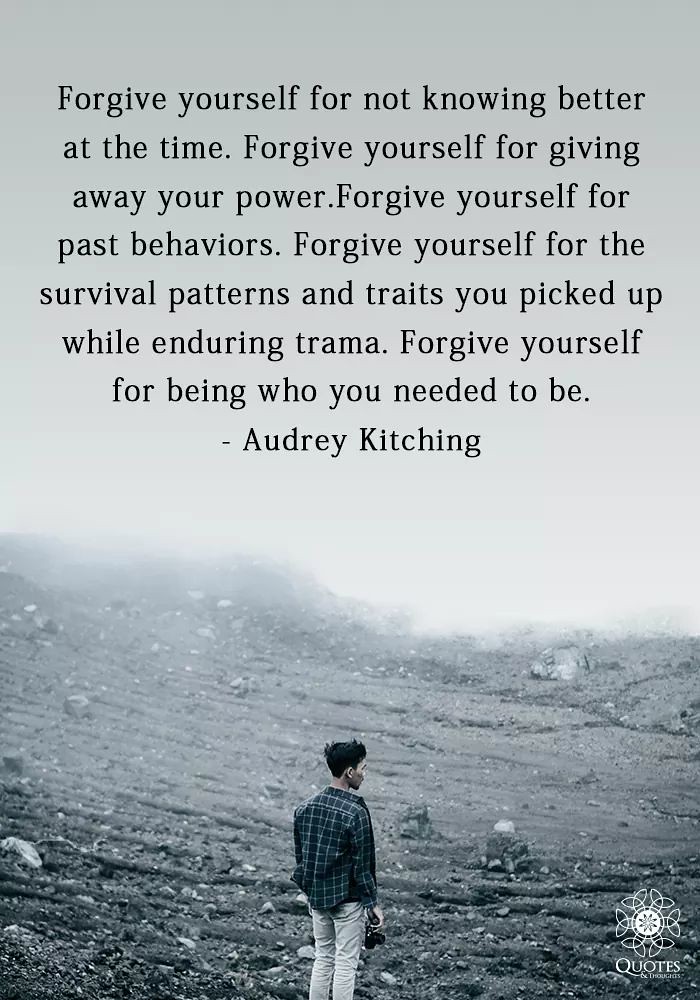This vertically aligned rectangular image, predominantly gray in color, depicts a solemn scene. The upper half of the image is a solid medium gray, representing a cloudy sky, transitioning to a lighter gray in the center, symbolizing a bright area amidst the overcast. The bottom half mirrors a darker gray, portraying a desolate landscape of grass interspersed with rocks and dirt. 

At the bottom center of the image stands a man, his back to the viewer. He wears a blue and white plaid long-sleeve button-down shirt and light-colored pants—either jeans or khakis. His short brown hair is partially visible. The man appears to be gazing over the barren terrain.

In the lower right-hand corner, a small logo features a flower inside a circle with surrounding petals, alongside the word "QUOTES" in white, capital letters. 

Centered at the top of the image, multiple lines of black text bear the following message: "Forgive yourself for not knowing better at the time. Forgive yourself for giving away your power. Forgive yourself for past behaviors. Forgive yourself for the survival patterns and traits you picked up while enduring trauma. Forgive yourself for being who you needed to be." This poignant quote is attributed to Audrey Kitching.